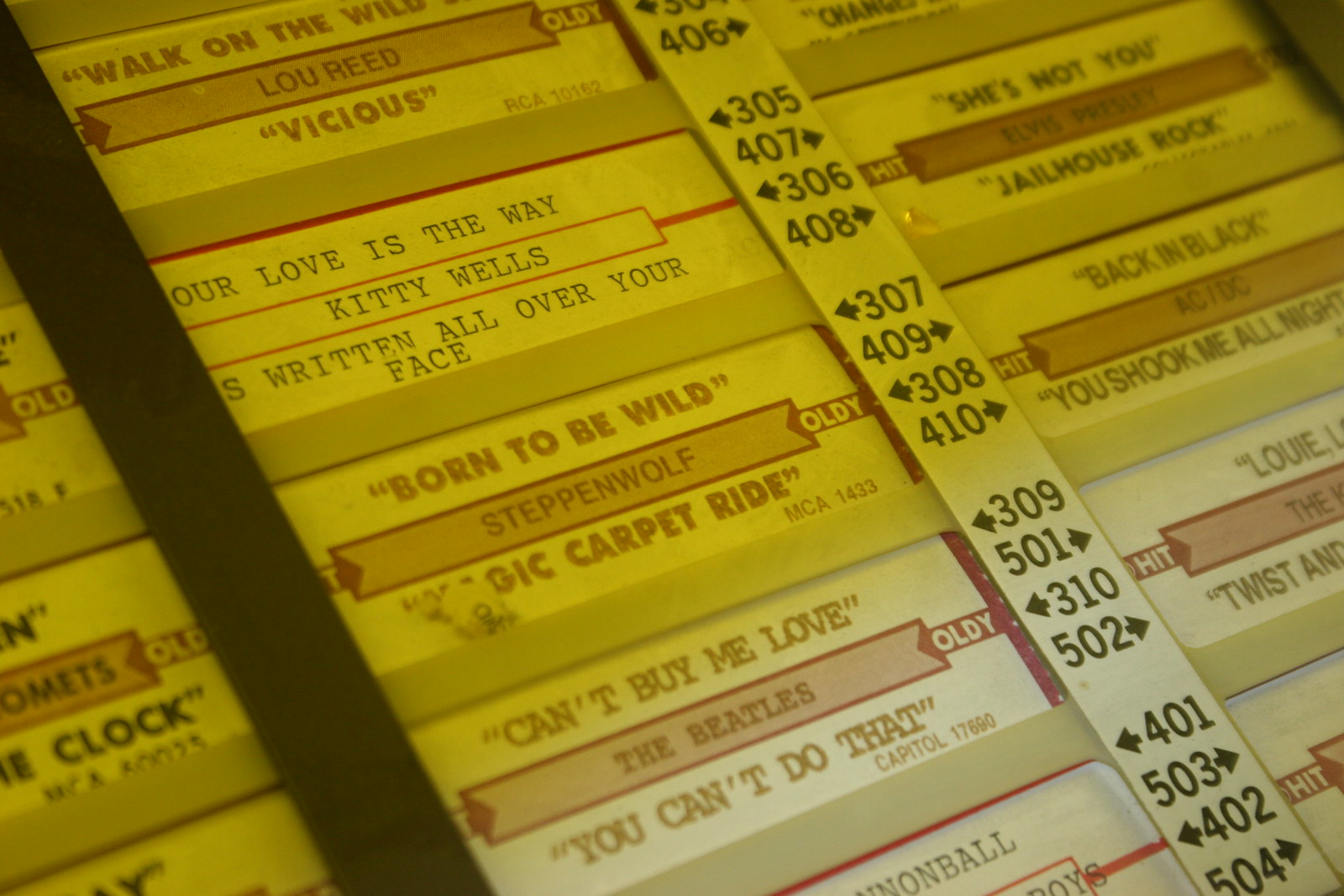The photograph captures a colorful jukebox interface showcasing a selection of classic songs and their corresponding artists. Prominently displayed are tracks like "Walk on the Wild Side" and "Vicious" by Lou Reed, "Our Love Is the Way" and "Written All Over Your Face" by Kitty Wells, and Steppenwolf’s "Born to Be Wild" and "Magic Carpet Ride." Classic Beatles hits "Can't Buy Me Love" and "You Can't Do That" are also visible, alongside AC/DC's "Back in Black" and "You Shook Me All Night Long." Elvis Presley's legendary "Jailhouse Rock" is listed as well. Each song is accompanied by the musician’s name, with tags such as "oldie" or "hit," and a number code, presumably for selection. The meticulously organized interface suggests a nostalgic musical journey, inviting listeners to select and enjoy timeless tracks.